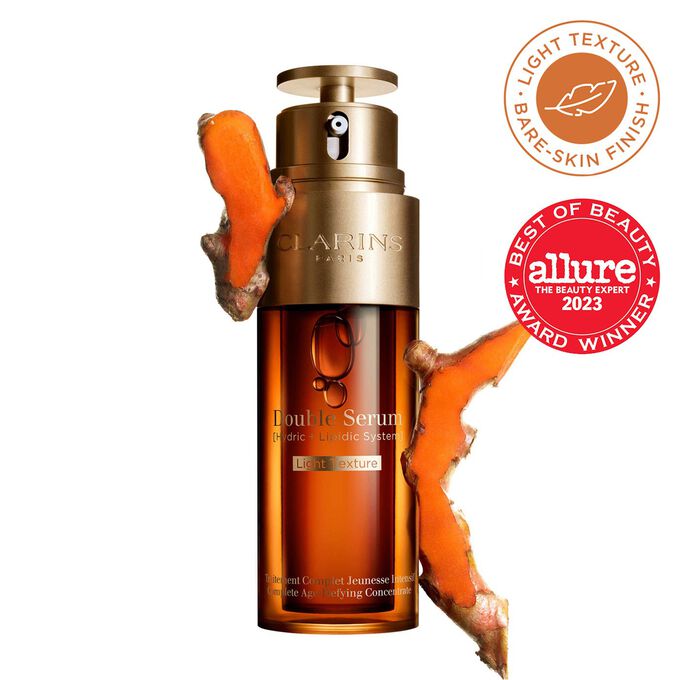The image is an advertisement for Clarins Paris Double Serum, featuring a pump bottle prominently displayed. The bottle, which is amber brown with a gold pump top and clear plastic casing, showcases gold lettering that reads "Clarins Paris Double Serum Hydric + Lipoic System." A gold banner accentuates the text "Light Texture." The bottle contains a deeper amber brown liquid with visible large bubbles trapped near the top, highlighting the dual-chamber design of the container. 

The base text, though mostly illegible, can be identified by reflection as stating "Age-Defying Concentrate." Accompanying the bottle are sliced cross-sections of turmeric root, adding a natural ingredient touch to the scene. On the right side of the image are two round labels. The top label, in coppery gold text, reads "Light Texture, Bare Skin Finish," along with a stylized leaf emblem. The bottom red label announces the product's accolade, "Best of Beauty Award Winner Allure The Beauty Expert 2023."

This combined detailed description captures the essence and highlights of the Clarins Paris Double Serum advertisement.